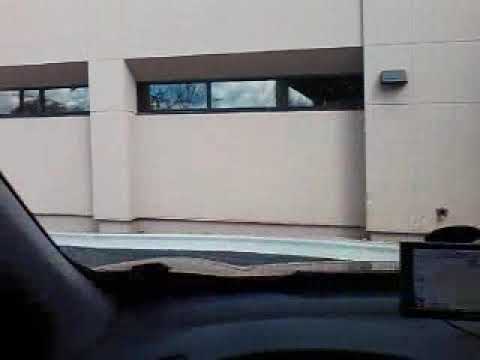The photograph, taken from within a dark green car, prominently features its dashboard and the lower portion of its interior, which is noticeably dark black in color. A GPS or mobile phone is mounted to the bottom right side of the windshield. Through the front window of the car, we can see the exterior of a cream-colored building with a turquoise base. The building features several rectangular-shaped glass windows reflecting the sky and trees, hinting at an outdoor setting during the middle of the day. The image composition primarily includes the building façade and windows positioned towards the top left, the dashboard at the lower part, and the GPS device in the bottom right corner. The overall scene shows the perspective from someone parked in front of the building, capturing a simple yet vivid moment without any text present in the image.